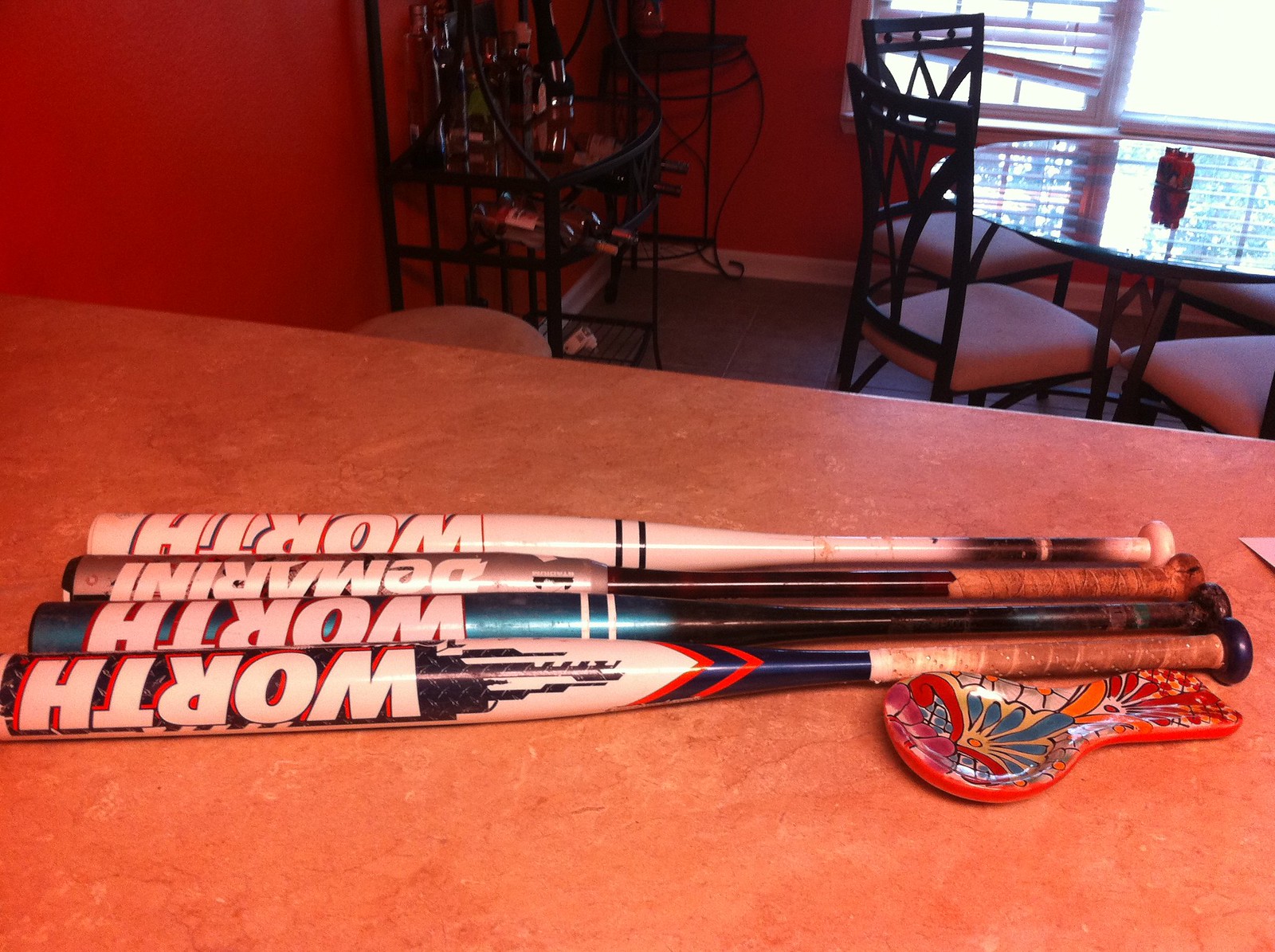This image features four decorated baseball bats laid out on a reddish-brown kitchen countertop inside a home. Three of the bats display the word "WORTH," while the third bat is branded "DEMARNI." The first bat is blue with an orange V-shape design and a white section with a black background. The second bat is metallic blue with a black handle, the third bat has a black handle and a silver top, and the fourth bat features a black and white handle. To the right of the bats' handles, there's a colorful spoon rest with psychedelic patterns, likely used next to a stove. In the background, a glass dining room table with a black iron base is surrounded by four padded chairs. A blue-lit area can be seen through a nearby window, and a black metal cabinet holding alcohol is positioned against the wall.